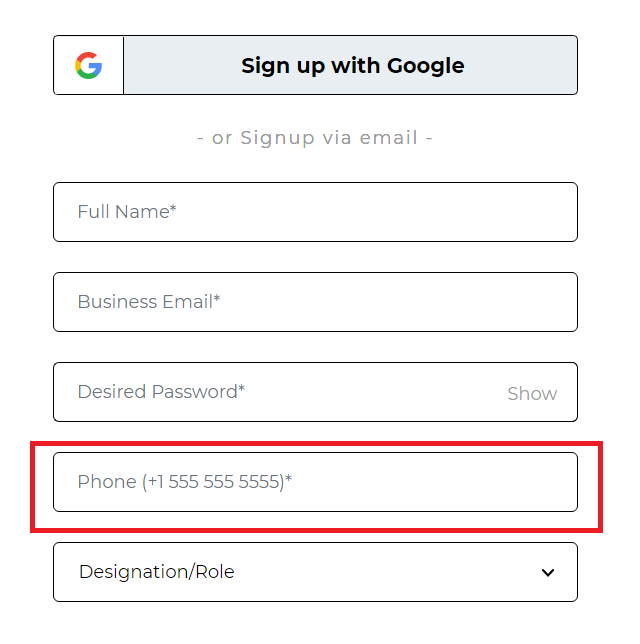The image displays a sign-up page for an unspecified service. At the top, a gray bar features the option to "Sign Up with Google" in bold, black letters next to Google's multicolored 'G' logo. Below this, light gray text offers an alternative to "Sign up via email."

The form includes several fields with white backgrounds and black borders. The first field requests the user's "Full Name," marked with an asterisk to indicate that it is required. Next, a similar field asks for a "Business Email," also required. Below this, another box for a "Desired Password" is provided, with an option to show the password. 

The following field for "Phone" is distinctly highlighted with a red, bold border and includes an example phone number, indicating its importance. Lastly, a field labeled "Designation/Role" includes a drop-down arrow for users to select their role. All required fields are marked with asterisks.